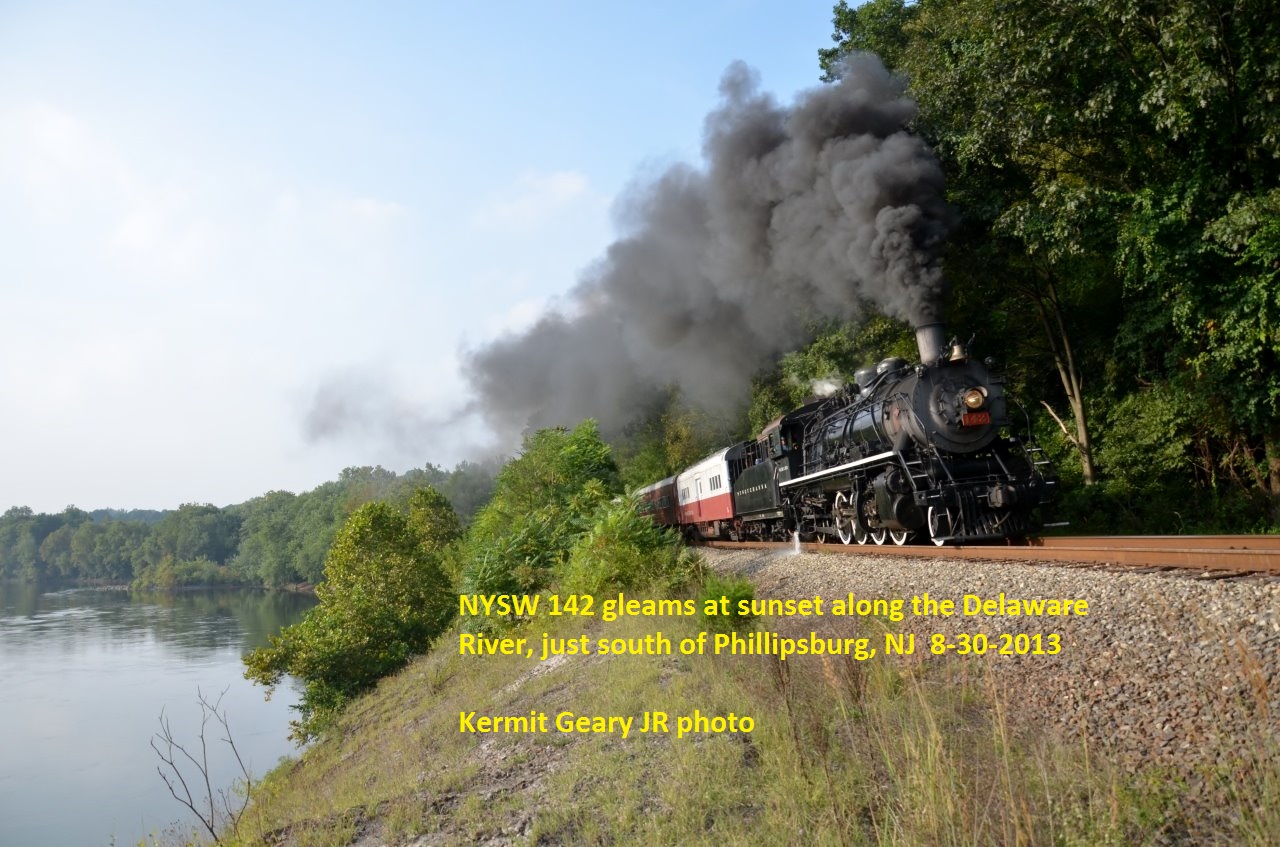The image captures an outdoor scene featuring a vibrant landscape with a steam engine train and accompanying text. At the center of the image, the black train, identified as NYSW 142, is seen barreling down rusted brown tracks toward the middle right, emitting a robust plume of dark gray smoke that envelops the top center of the image and merges with the partly cloudy sky. This steam engine train has a black front with red and white cars trailing behind. Flanked by lush green trees on the right and bordered by a downhill incline leading to a bluish-gray lake on the bottom left, the scene is a picturesque mixture of natural and manmade elements. The background, especially towards the left side, showcases additional green trees beneath a sky that transitions from white and blue to gray. Superimposed at the bottom center in yellow font are the words: "NYSW 142 gleams at sunset along the Delaware River just south of Phillipsburg NJ 8-30-2013. Kermit Geary JR Photo."